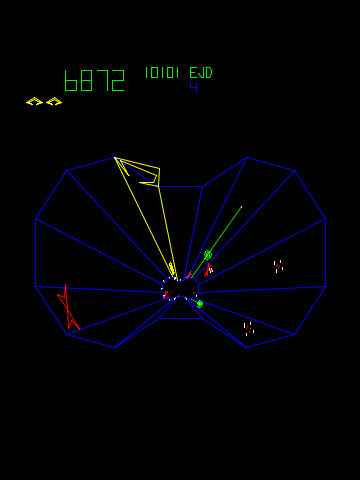The image captures the screen of a retro-style video game, characterized by its primitive graphics. Against a solid black background, the top of the screen prominently displays two yellow icons, which likely represent the player's remaining lives. Following that, bold green numbers indicating a score of 6872 are displayed, with an additional set of green characters "10101 EGD" to the right and a blue number "4" below it.

Dominating the middle of the screen are intricate blue lines radiating from the center to form a complex pattern resembling a series of triangles creating a circular design. Within this pattern, a yellow oval sits in the center, intersected by various geometric shapes: a red triangle on the left, a diagonal green line, and two long neon yellow lines stretching to the edges. Scattered around are smaller colored shapes, including two small red circles with white dots, possibly representing enemies moving in from the right side. The visual aesthetic is similar to classic games like Pac-Man, but with an array of colorful lines creating a more chaotic, dynamic environment.